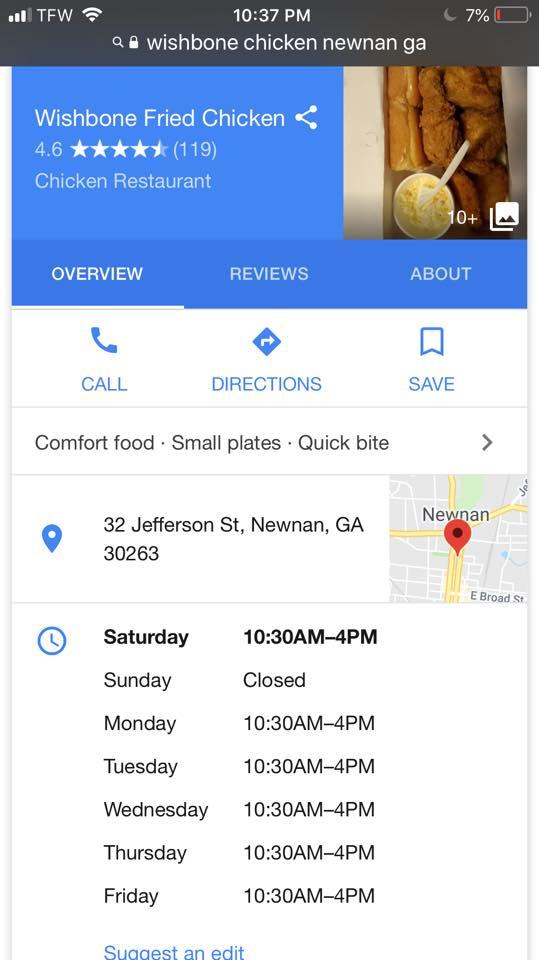Screenshot of a listing for Wishbone Fried Chicken in Noonan, Georgia. In the upper right-hand corner, there is an image of a meal featuring a box with crispy chicken, bread, and a small side dish served in a white bowl. Beside this photo, white text indicates "10+" accompanied by an icon representing that there are 10 additional photos of the restaurant or its food. To the left, a blue rectangle with white text displays, "Wishbone Fried Chicken, 4.6 out of 5 stars, based on 119 reviews." This section also includes the labels "Chicken Restaurant" and tabs for "Overview," "Reviews," and "About."

Below this, three clickable icons on a white background offer options labeled "Call," "Directions," and "Save." Further down, a small square map with a red location pin highlights the restaurant's position in Noonan. At the bottom, the restaurant's operating hours are displayed, spanning from Saturday through Friday.